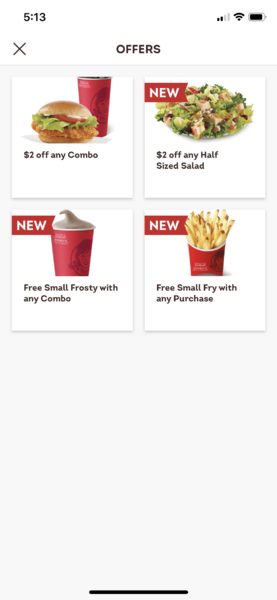A screenshot of a mobile phone displaying promotional offers from Wendy's. The top part of the screen shows the time "5:13" in black print, along with Wi-Fi, signal bars, and a nearly full battery icon. Below that, the top of the app screen has a blackish-brown "OFFERS" label in all capital letters with an "X" on the left. The main content includes various promotional deals: 

1. On the left, an image of a chicken sandwich with lettuce and tomato, accompanied by a drink in the background, advertises "$2 Off Any Combo."
2. On the right, a salad with chicken pieces, onions, and other vegetables is highlighted with a red banner saying "NEW" in white letters, offering "$2 Off Any Half-Sized Salad."
3. The bottom-left section features an offer for a "Free Small Frosty with Any Combo" under a "NEW" banner.
4. The bottom-right shows an image of fries with a "NEW" banner, promoting a "Free Small Fry with Any Purchase."